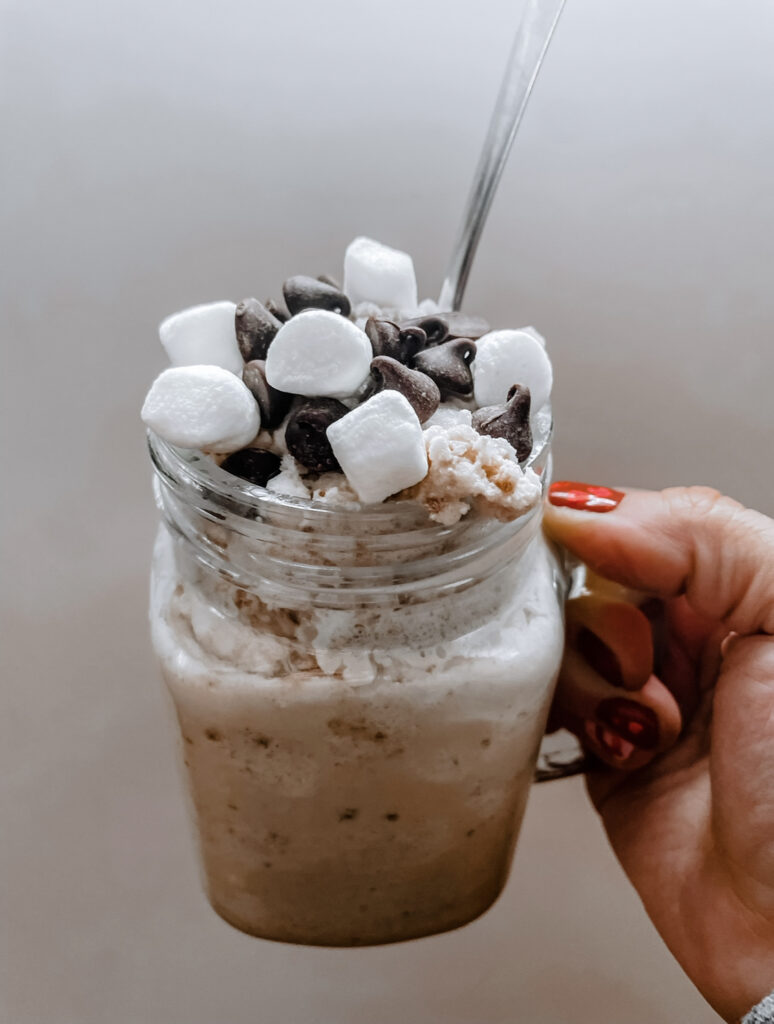The image depicts a close-up of a clear mug, resembling a mason jar with a handle, held by a person with red nail polish. The gradient background transitions from light gray to purplish gray. The jar contains a light brown beverage, likely an iced coffee or chocolate frappe, which darkens toward the bottom. Atop the drink is a generous dollop of whipped cream, drizzled with chocolate, and adorned with tiny marshmallows, chocolate chips, and possibly a walnut. A silver spoon is seen protruding from the top. The focus of the image is mainly on the mug and its rich, sweet contents, with no other text or identifiable background elements.